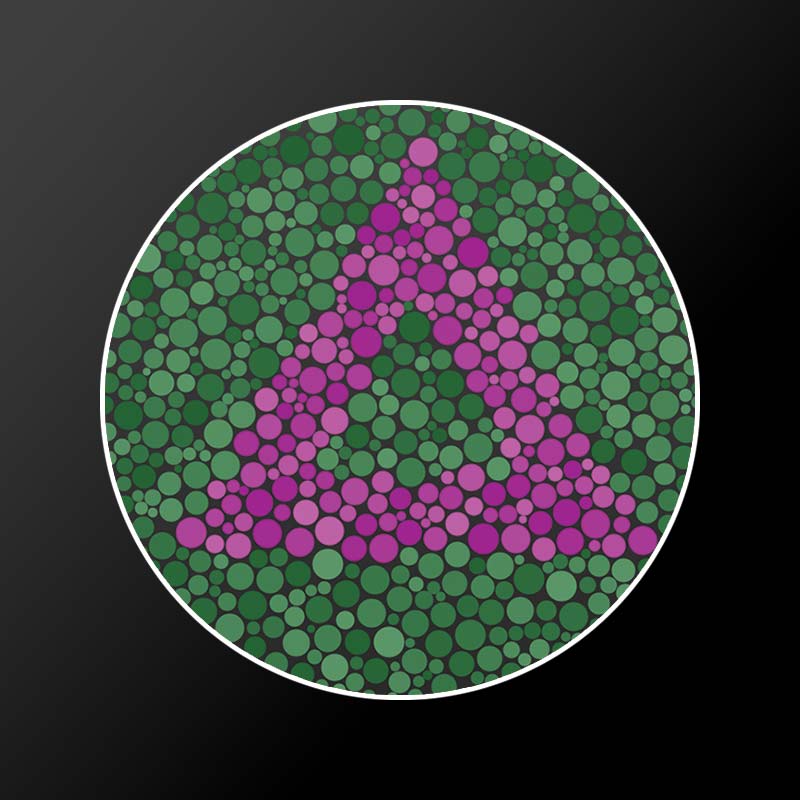This image is a nearly square rectangular piece primarily featuring a prominent white-outlined circle in its center. The background outside the circle gradiates from black on the right side to gray on the left. Within the white circle, a myriad of colorful dots of varying sizes create a detailed pattern against a dark gray backdrop. Most of these dots are shades of green, forming a broad area. In the middle of this green expanse is a large purple triangle pointing upwards, nearly spanning the circle's width but stopping just short of the left edge while touching the right edge. Nestled within the purple triangle is a smaller green triangle. This intricate arrangement of dots forms a visual reminiscent of a color blindness test.